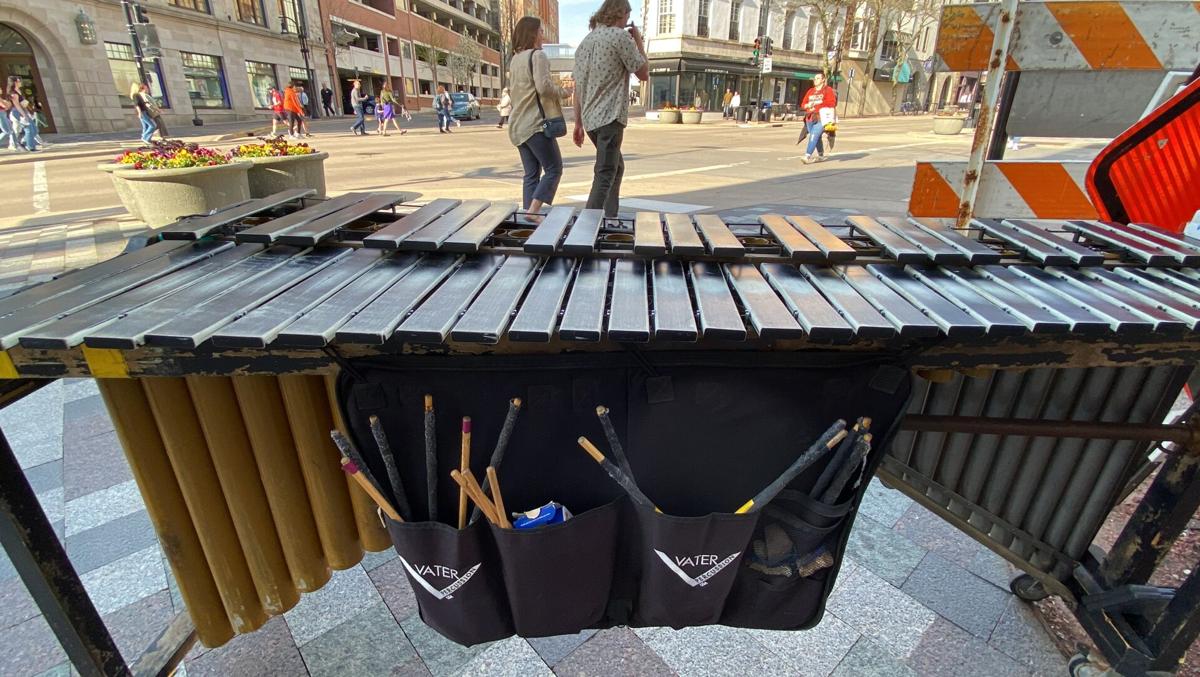The photo vividly captures a bustling city street corner, where a street musician's xylophone, prominently featuring black keys and yellow-gray pipes, occupies the foreground. The musician's black pouches, brimming with drumsticks, hang from the instrument, which is situated near a busy intersection. People, both men and women, can be seen crossing the streets and walking on the sidewalks, enveloped by the energy of the city. Nearby, colorful flower pots—adorned with yellow, green, and magenta blooms—decorate the sidewalk. Many buildings and a parking garage frame the background, with cars navigating the roads. Sunlight bathes the scene, highlighting construction signs and details of this vibrant urban landscape from the eye level of the street performer.